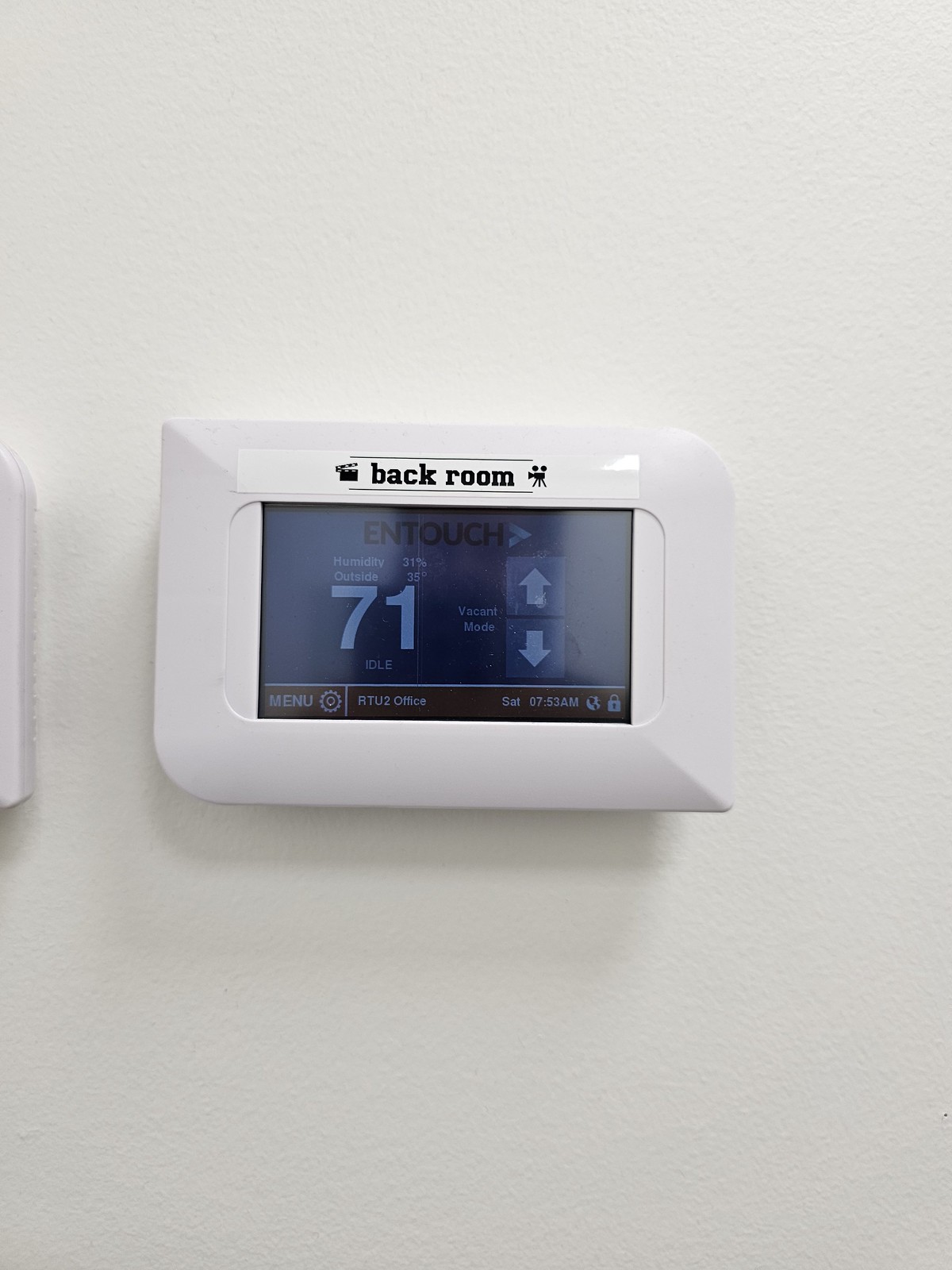The image features a close-up of a white wall with a temperature thermostat prominently centered. This thermostat has a digital display and is housed within a white, landscape-oriented rectangular plastic frame that has contrasting pointed and curved corners—the upper left and bottom right corners are pointed, while the upper right and lower left corners are curved. Above the LED display, a white sticker with the words "Back Room" written in black is adhered to the housing.

The LED screen itself has a dark blue background with a brown chiron at the bottom. The brown chiron features white text, with "Menu" displayed on the bottom left and the current date and time on the bottom right. The upper section of the screen showcases a large number "71," indicating the current temperature, and is flanked by large white arrows pointing up and down, which likely serve as controls to adjust the temperature.